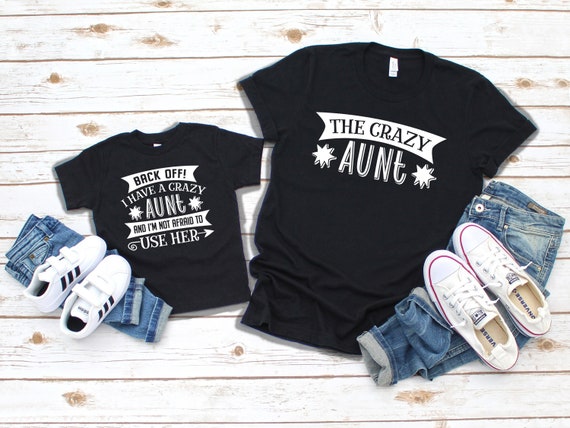The image shows a coordinated outfit set displayed on a white wood floor with visible brown knots and grain running horizontally. On the right side, there is an adult-sized black t-shirt bearing the text "The Crazy Aunt" in white, accented with stars around the word "Aunt." Below this t-shirt, a pair of blue jeans are neatly folded with a white pair of Converse sneakers featuring a red outline at the toes placed on top. 

To the left, the matching set for a child is arranged. The child-sized black t-shirt reads: "Back Off, I Have a Crazy Aunt, and I'm Not Afraid to Use Her," with an arrow pointing towards the notion of the aunt. This t-shirt also includes star accents similar to the adult version. Beside this t-shirt, there's a pair of folded blue jeans, topped with white sneakers that have black stripes over the Velcro closures.

The items are organized in a visually appealing manner, with the children's outfit on the left and the adult's outfit on the right, showcasing a matching ensemble perfect for a fun and coordinated look.